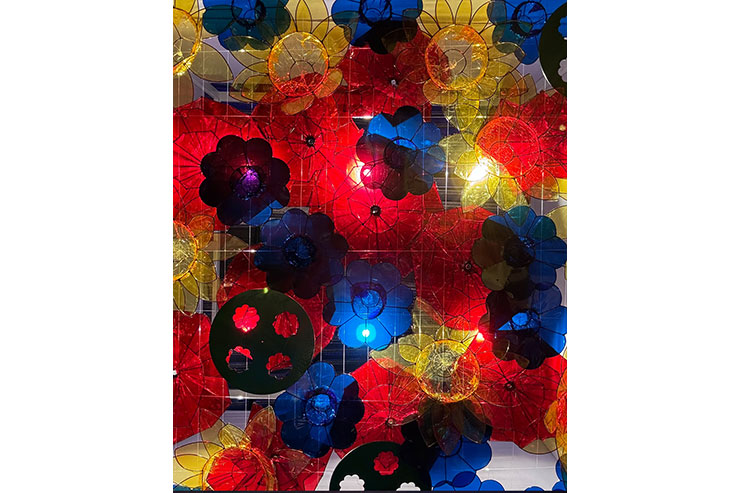This detailed color photograph showcases a stunning piece of modern, psychedelic, fractal art. The artwork primarily consists of intricately designed flowers crafted from colored cellophane, giving them a translucent quality. The flowers are predominantly blue, red, and yellow, and are connected in a complex, almost fractal pattern, with petals featuring various angles. These flower shapes, likely suspended from a ceiling by delicate white filaments, are illuminated by points of light from the center right area, making them glow ethereally. 

A striking feature in the composition is a solid black disc with flower-shaped holes, through which the floral decorations and lights shimmer. The foreground is dominated by the vivid blue flowers, while the background features what appear to be red, open-umbrella-shaped decorations, enhancing the piece’s dimensionality. The layered arrangement of the flowers, with blue overlapping red and red overlapping yellow, adds to the rich depth of the visual experience. This artwork, combining light, color, and intricate design, emanates a mesmerising, almost otherworldly beauty.